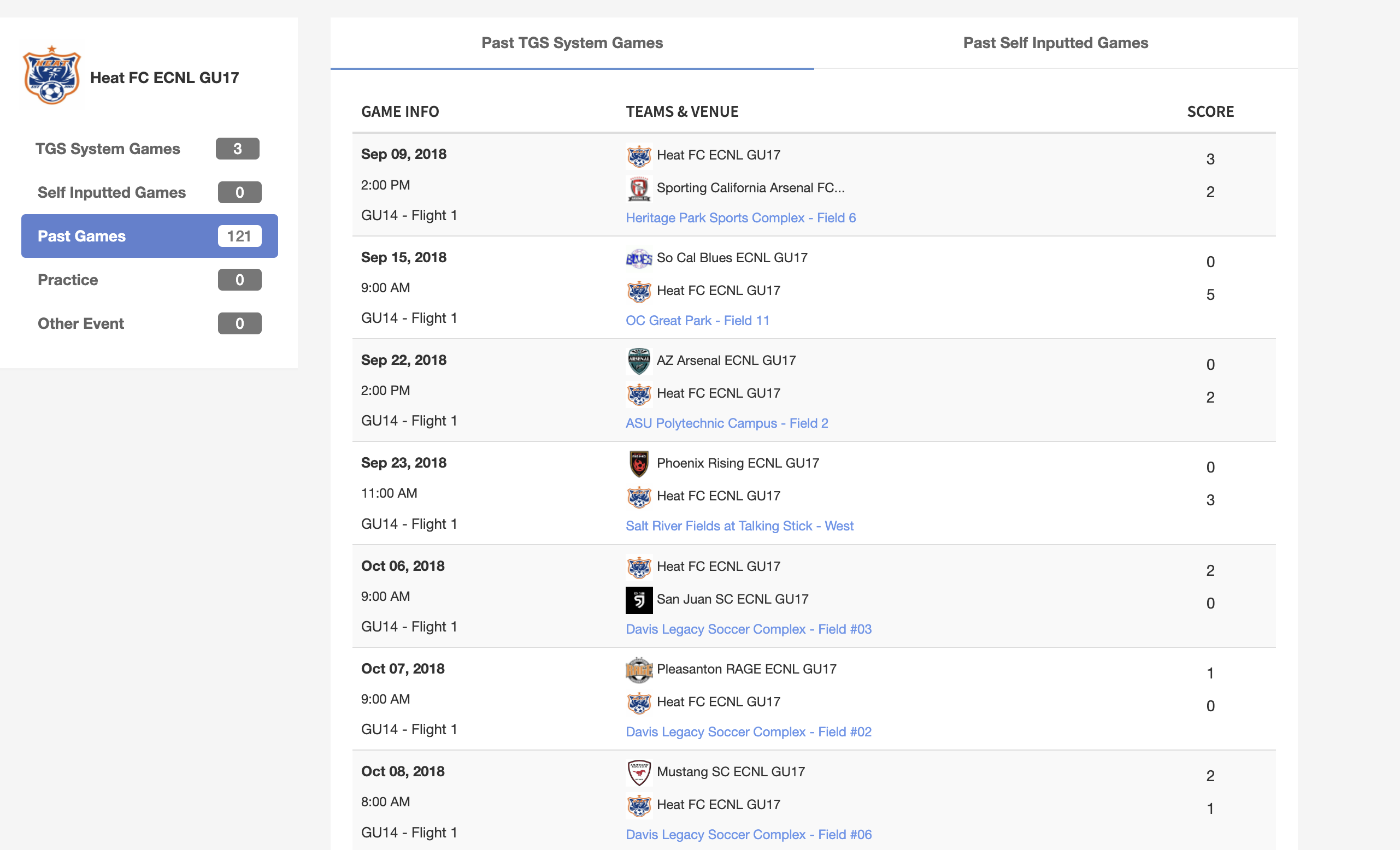The image showcases a section of a sports team's website, specifically dedicated to Heat FC's ECNL GU17 soccer team. Prominently displayed in the top left corner is the team's emblem, featuring a soccer ball, indicative of their sport. Adjacent to the emblem is a red box containing navigational options labeled "TGS system games," "self-inputted games," "past games" (highlighted in blue), "practice," and "other event" (in black). 

On the right side, there is a detailed schedule displayed in a tabular format. The chart is categorized under headers such as "Past TGS System Games" and "Past Self-Inputted Games," organized in a vertical layout. Each entry provides comprehensive game information, including date, time, venue, and opposing team. For instance, the first recorded game is dated September 9, 2018, featuring a 2 p.m. match between Heat FC and Sporting California Arsenal. The schedule spans matches up until October 8, 2018, with details about the outcomes for each game.